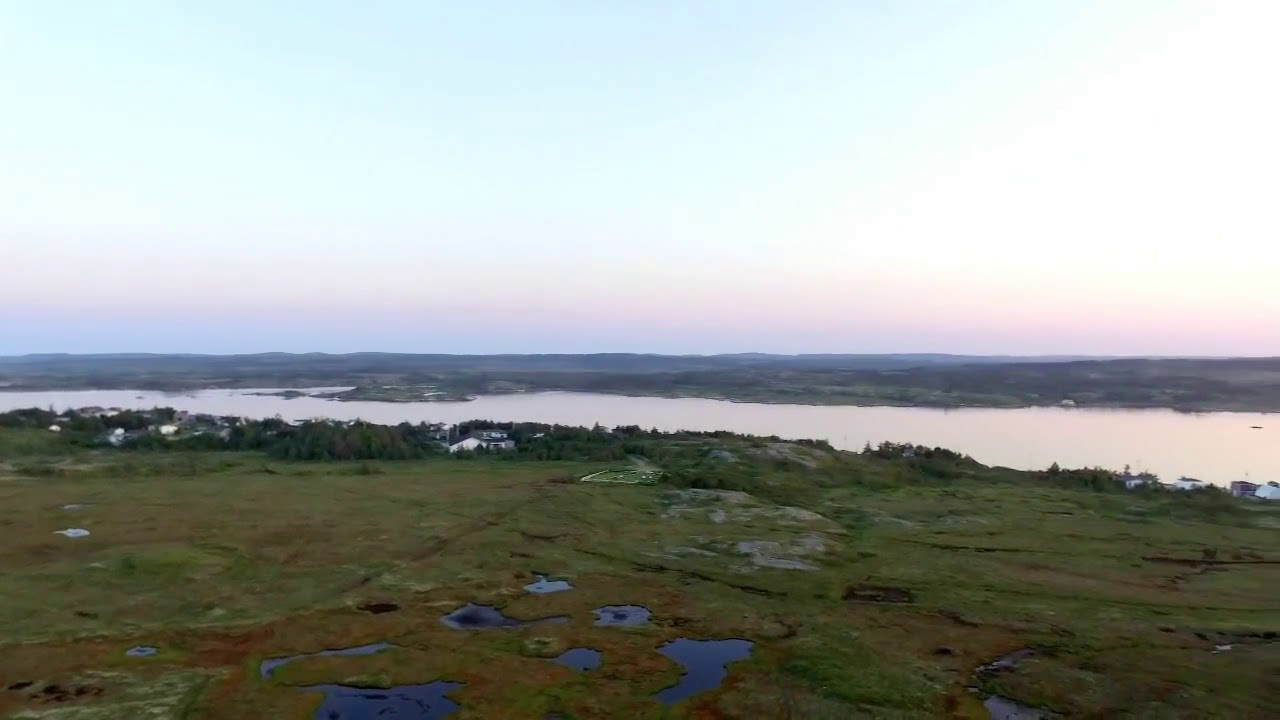The aerial photograph captures a vast, desolate marshland during the daytime, featuring a combination of weathered green fields interspersed with numerous water deposits and ponds. The foreground showcases a marshy plain with grass that appears heavily worn, possibly by tractors or storms, adding a textured, rugged look to the landscape. In the center of the image, a highly illuminated river, almost white due to the reflection of sunlight, horizontally divides the scene, creating a natural boundary between two landmasses. Scattered houses can be seen along the river's edge, emphasizing the area's sparse development. The background comprises a thin strip of mountain ranges or hilltops under a clear, light blue sky. A delicate, thin cloud stretches from the center-left of the image towards the upper right-hand corner, adding subtle detail to the serene skyline, tinged with soft hues of pink, orange, and yellow suggesting the early morning light.